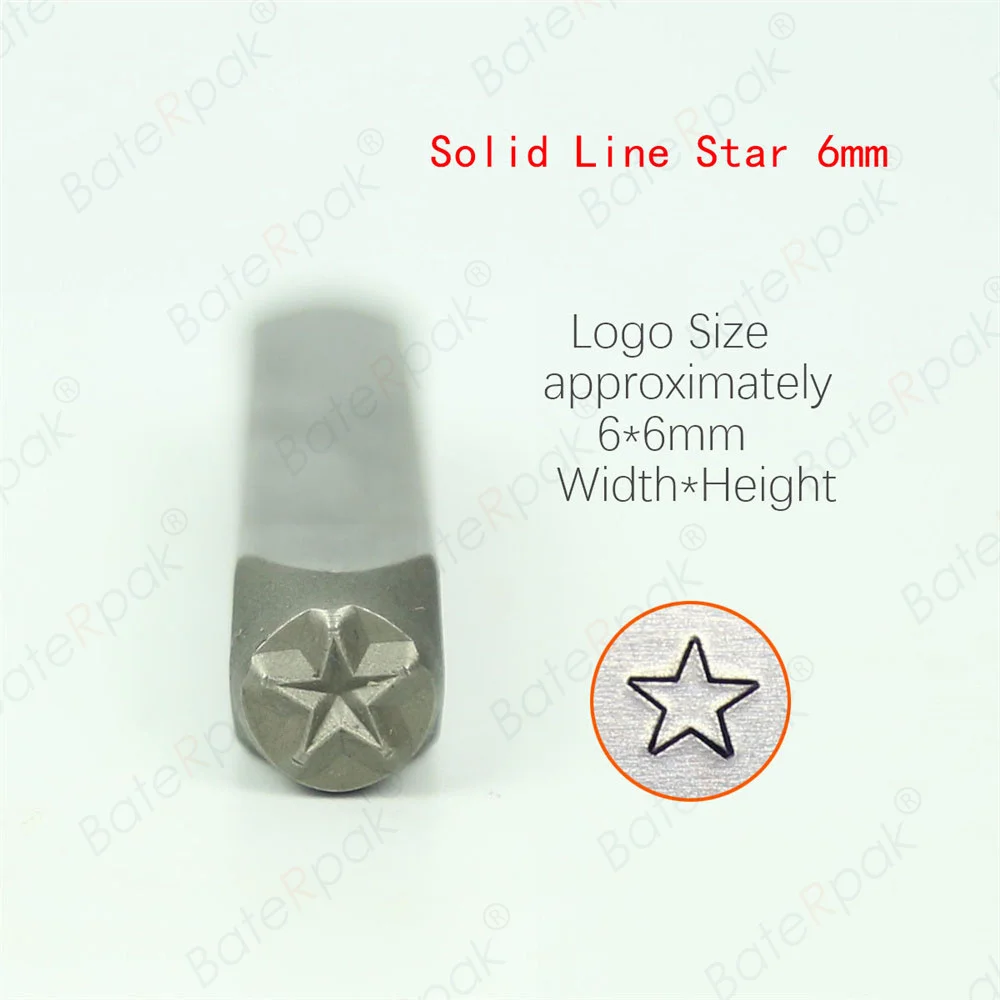The image depicts a detailed digital poster with a light teal background, heavily overlaid with repeated gray watermarks reading "Bait or Peck." At the top right, bold red text states "Solid Line Star 6mm" followed by the description "Logo size approximately 6 star 6mm width x height." Below this text lies a drawing featuring a circular shape filled with gray, outlined in red, and containing a prominent black, five-sided star. Adjacent to this on the left is a metallic, dark gray object resembling a microphone, matching the shape of the drawing but with an orange circle encasing another black star. The image is visually dense, merging textual descriptions with emblematic graphics.